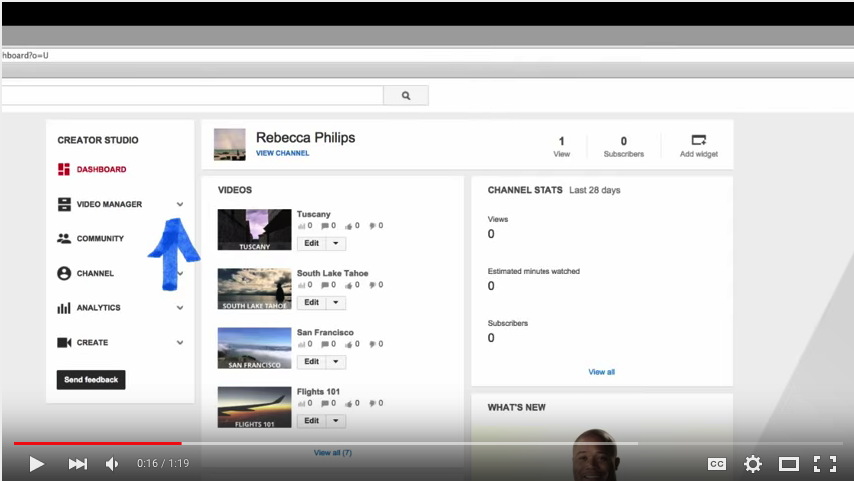A screenshot of a website displays a partially visible URL in the address bar, reading "dashboard/o=u." Below the address bar, there is a search bar and a search button indicated by a magnifying glass icon. The main content of the page appears to be a profile interface for a creator studio. The sidebar on the left features a vertical menu with the following options: Dashboard, Video Manager, Community, Channel, Analytics, Create, and a Send Feedback button at the bottom.

In the center of the page, the name "Rebecca Phillips" is prominently displayed with a corresponding profile picture and a blue hyperlink beneath the name that reads "View Channel." To the right of the name are indicators showing "1 view," "subscribers," and an "add widget" option.

Below Rebecca Phillips' name, the middle section of the page lists several video titles: "Tuscany," "South Lake Tahoe," "San Francisco," and at the bottom, "Flights 101." On the right side of the page, a vertical list labeled "Channel Stats" provides performance metrics for the last 28 days, showing "views: 0," "estimated minutes watched: 0," "subscribers: 0," and a section titled "What's New."